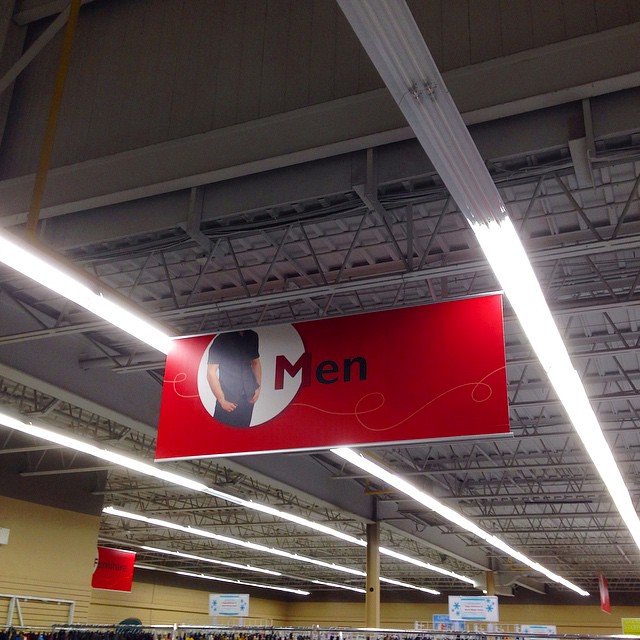In this photograph taken inside a department store, you immediately notice the high ceilings, which showcase an industrial aesthetic with visible metal supports and rafters. The ceiling is adorned with diagonal strips of fluorescent tube lighting that illuminate the space. The lower portion of the walls is painted a yellow hue, while the upper section above the lights features a gray and tan palette.

Prominently displayed in the image is a solid red rectangular sign with a white decorative curved line sweeping across it. Centrally placed on the sign is a circular emblem with a white background, inside of which is the figure of a man dressed in black shirt and pants, symbolizing the men's section. The word "men" is written in bold, with the letter "M" in red and the "E" and "N" in black. This clean and vivid signage guides shoppers towards the men's clothing area in the store.